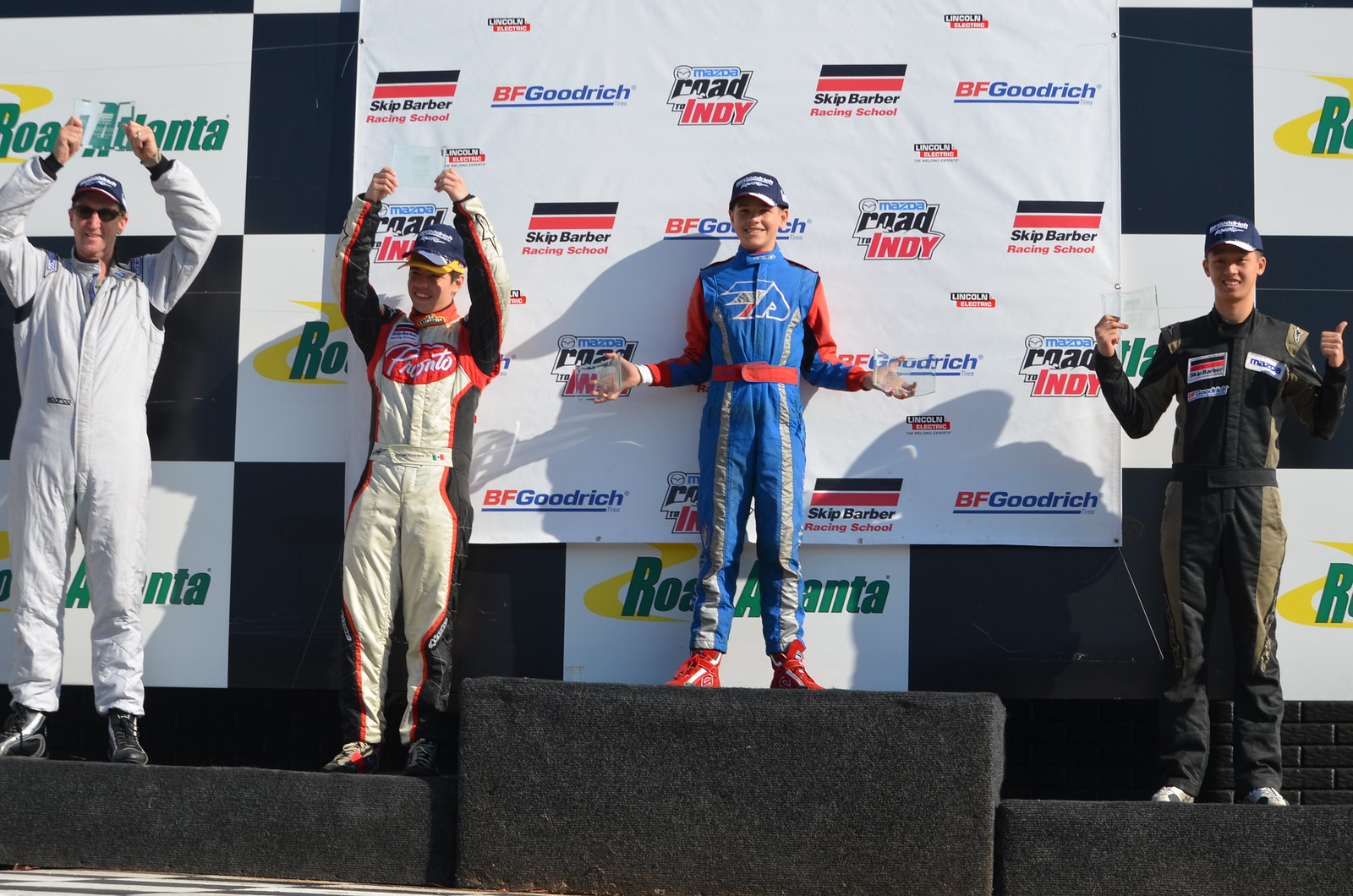In the photograph, four individuals are standing on a podium with positions marked from first to fourth, celebrating what appears to be a racing championship. The background features a banner adorned with the logos "BF Goodrich," "Mazda Road to Indy," and "Skip Barber Racing School." Central to the image is a young boy in a blue racing jumpsuit standing on the tallest podium, his arms extended holding a clear glass award in each hand. To his right and slightly elevated is another boy in a black racing suit giving a thumbs-up while also holding a glass award. To his left is a youngster in a white and black jumpsuit, also with an award in hand. Additionally, on the far left, there's an adult man in sunglasses and a ball cap wearing a white racing suit, holding a glass award. The boys’ outfits and the awards they hold signify their achievements, while the arrayed podiums emphasizes their standings in the race.